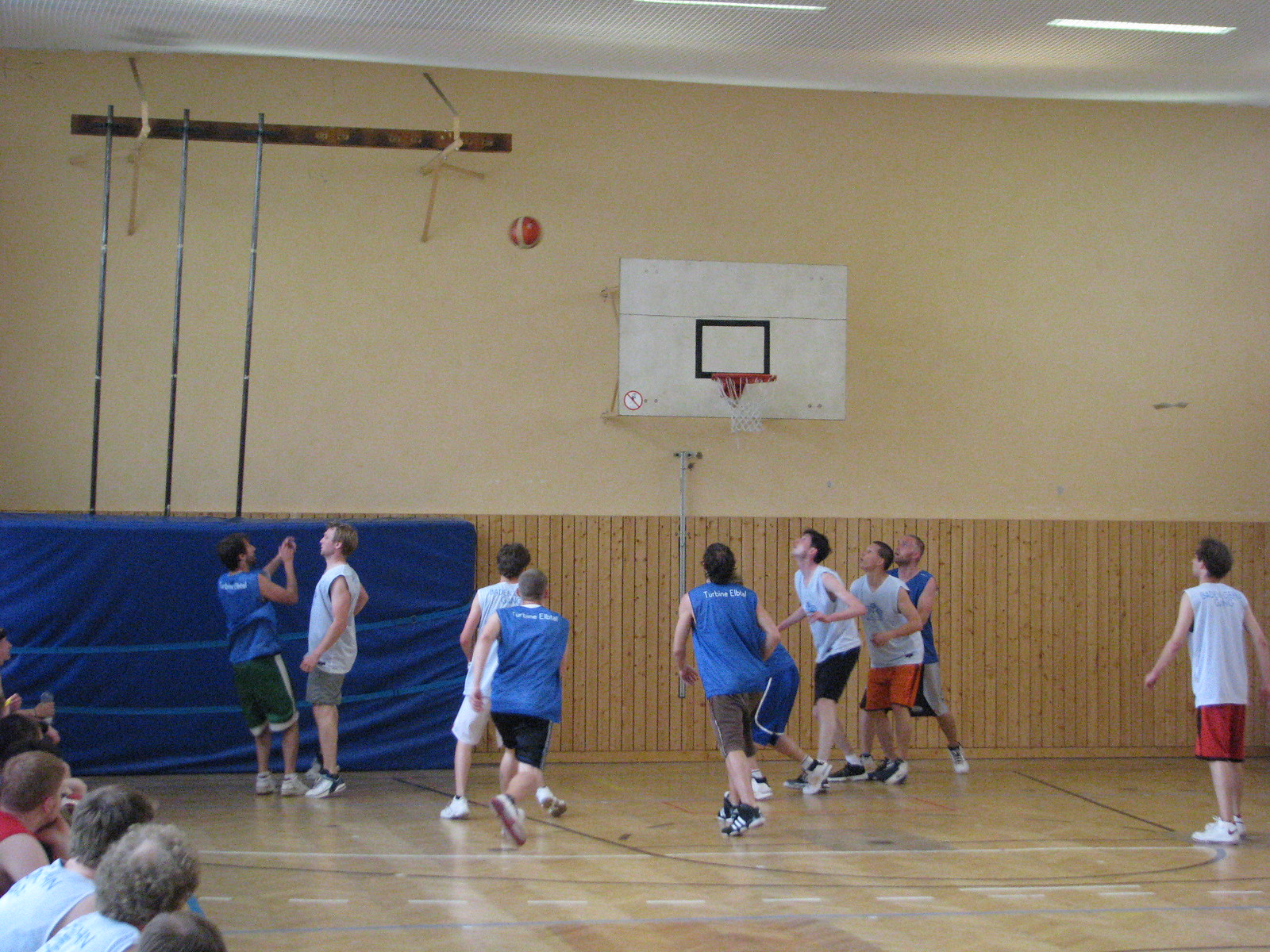This photograph captures the lively atmosphere of a local community center during an indoor basketball game. The well-loved basketball court, with its shiny surface and slightly dingy hoop, speaks to countless games played here. The beige walls, interspersed with darker vertical wooden panels, provide a modest backdrop. Rectangular, white lights hang from the ceiling, casting a bright light over the scene.

In the center of the image, a group of young boys, dressed in various colored shorts and tank tops, are engrossed in the game. One boy on the left side has just launched the orange and white basketball into the air. To the left, a blue-paneled section below some poles hints at makeshift features of the gym. Meanwhile, a crowd of excited spectators, seated and standing along the wall, keenly watches the action unfold, creating an engaging and heartwarming community atmosphere.